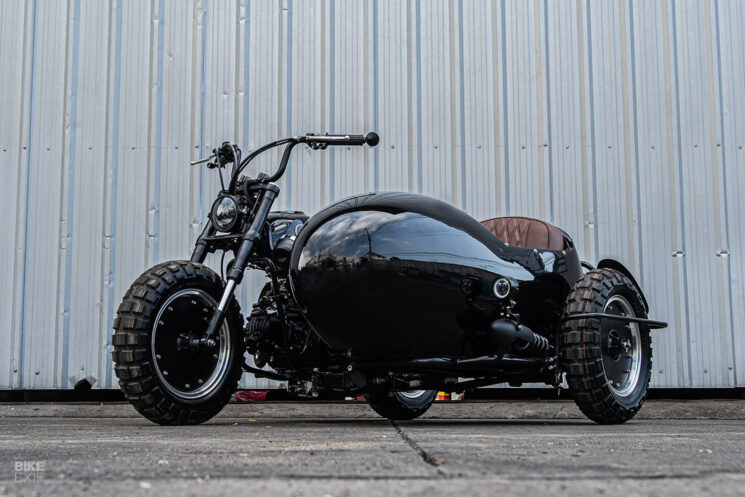In this ground-level outdoor photo, a unique black motorcycle with a matching sidecar is prominently featured in front of a corrugated metal wall that has vertical grading marks. The sidecar, attached centrally to the motorcycle, is a single-seater with a thick, brown leather cushion. The motorcycle and sidecar together have three wheels in total, each with shiny, textured black tires. The motorcycle is equipped with black handlebars on both sides, adding to its sleek appearance. A watermark reading "Bike XC EXIE or XF XE" can be seen at the bottom left of the image.